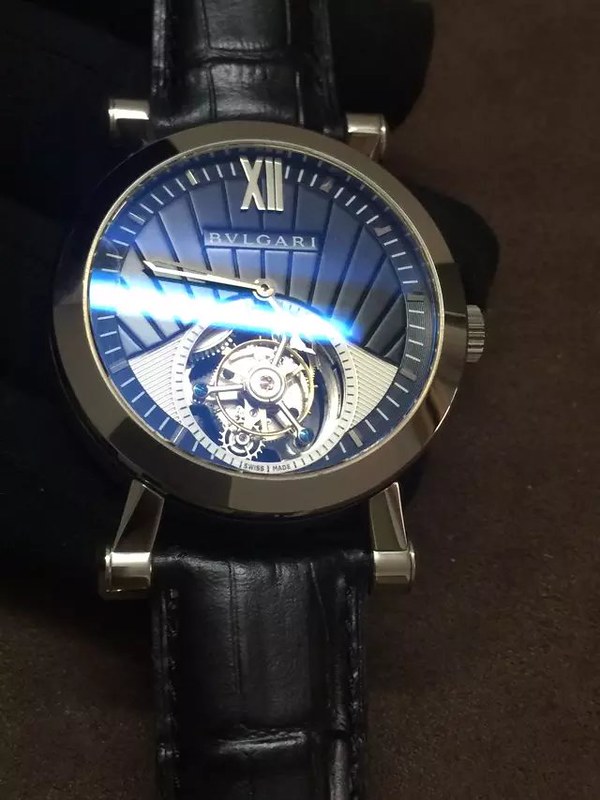This close-up photo showcases a sophisticated wristwatch against a white backdrop, with the image itself framed by a brown background. Although the entire watch isn't fully visible, the composition effectively highlights the central elements and a portion of the leather straps. The watch features sleek, black leather straps attached to a polished silver bar that seamlessly connects to the dial. 

Dominating the center, the watch face is encased in a silver frame, with a rich, blue interior detailed with fine lines radiating outwards, mimicking the appearance of a sunrise. Notably absent of numerals, the face highlights the 12 o'clock position with a silver Roman numeral XII. The hour markers are subtly denoted by darker notches, providing an elegant contrast. The minute and hour hands are crafted in silver, adding to the watch's refined aesthetic. An additional intricate sub-dial reveals a glimpse of exposed gears, showcasing the watch's mechanical intricacies and adding a layer of complexity to its design.